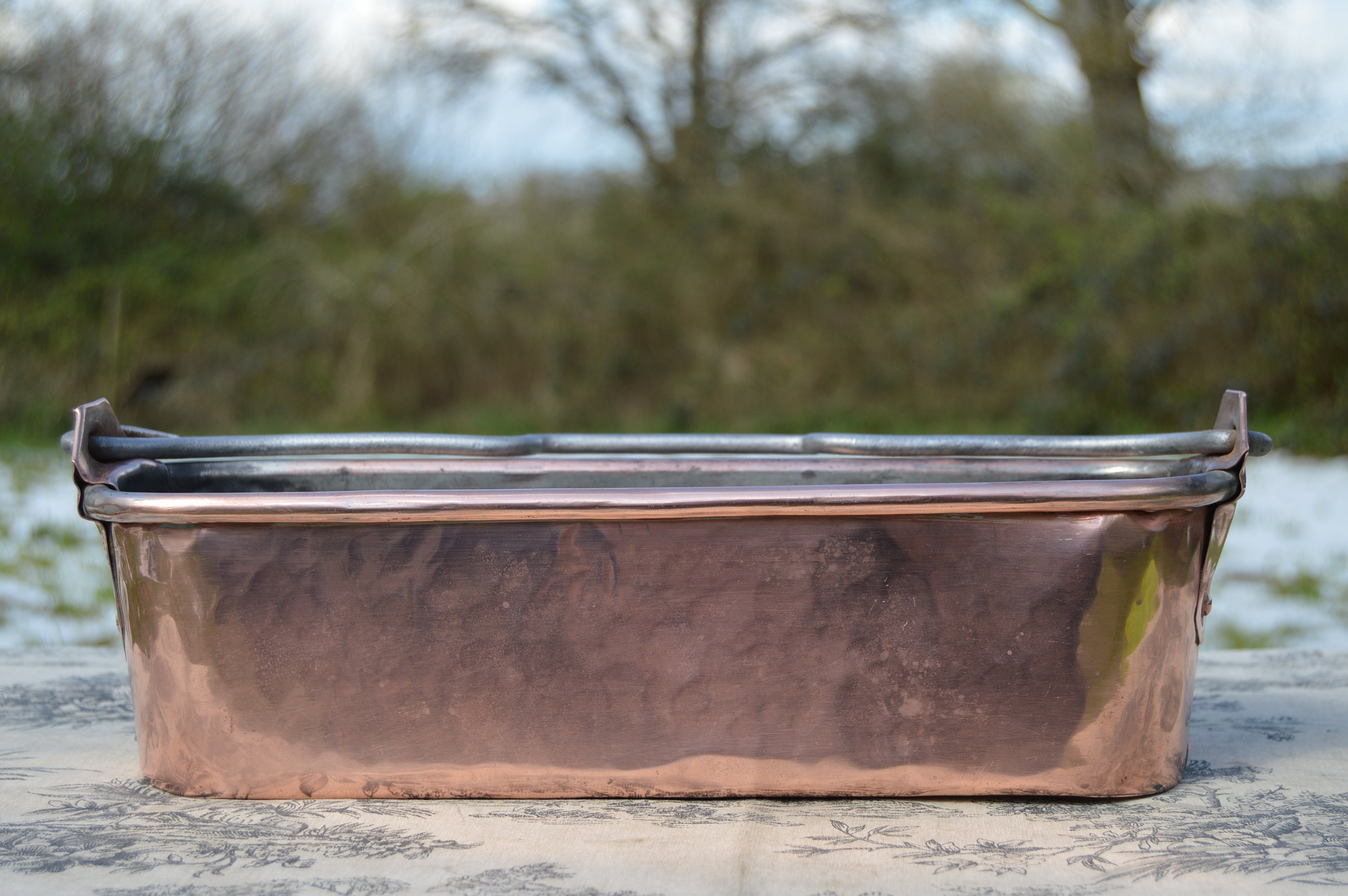The image depicts an outdoor scene featuring a table adorned with a white tablecloth patterned with scattered black flowers of varying heights. At the center of the table rests a metal tray with a copper-colored bottom and a silver-toned handle. The tray's handle is designed with a zigzag pattern and can be adjusted, featuring small latches on the sides. In the background, a sandy beach area is visible with patches of green grass and weeds growing through it. Further beyond, an expanse of shrubs and bare-branched trees extends into the distance, all under a slightly blurred blue sky. A tree trunk is noticeable in the upper right corner, adding to the rustic and natural setting of the scene.